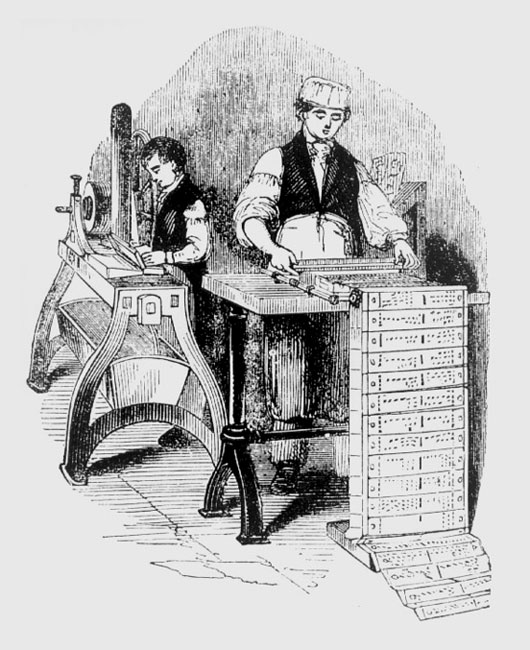The hand-drawn line art illustration, possibly created with an inky pencil on white paper, portrays an olden-day factory or workshop scene with two men busily engaged in their tasks. The background of the image is stark white, punctuated by inky spots, suggesting a richly textured and detailed composition.

On the right side of the drawing, a man is depicted with meticulous detail; he wears a white long-sleeved shirt with the sleeves rolled up to his elbows and a dark vest over it. His attire is completed with black and white pinstripe pants, a pillbox hat, and arm protectors. He appears to be operating a printing machine, his hands placed on it as sheets, possibly money or prints, emerge neatly onto the floor, covered in inky spots.

On the left, a younger man stands at a different, somewhat indiscernible machine, which has a cradle-like structure underneath. He is dressed similarly in a white shirt and dark vest but sans a hat. His hair is short, and he appears to be focused on his work. The machine he's operating could be a sewing machine or another type of equipment.

The detailed lines and textures in the drawing highlight the intense manual labor and intricate machinery of the period, successfully capturing a moment of industrious engagement in a historical setting.